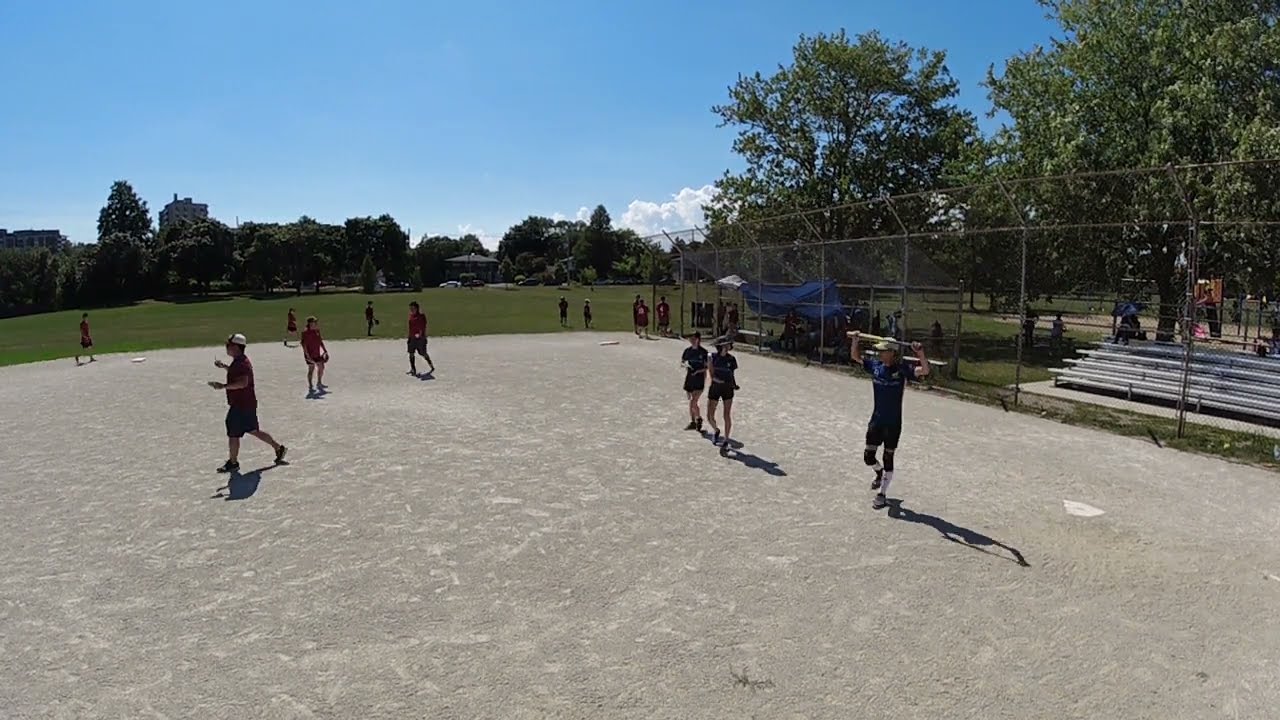The image depicts a baseball game set in a park with a dirt field. A home plate, first base, and second base are visible, though there are no marked lines to indicate the diamond. The field is surrounded by grass and a fence that separates the playing area from the bleachers on the right side, with a blue tarp covering a section of the stands. To the left, five men wearing red shirts and various color hats—white and black—are visible. In the center, two women dressed identically in black shorts, black t-shirts, black hats, and black shoes stand together. On the right side of the image, a player wearing knee pads holds a bat above their head, with hands positioned for a swing: one hand at the handle and the other at the bat’s end. The scene is set during a bright early evening, with shadows cast on the ground and a clear blue sky with clouds in the distance. The background features a green field, trees, and a tall building on the left side, indicating an urban environment.